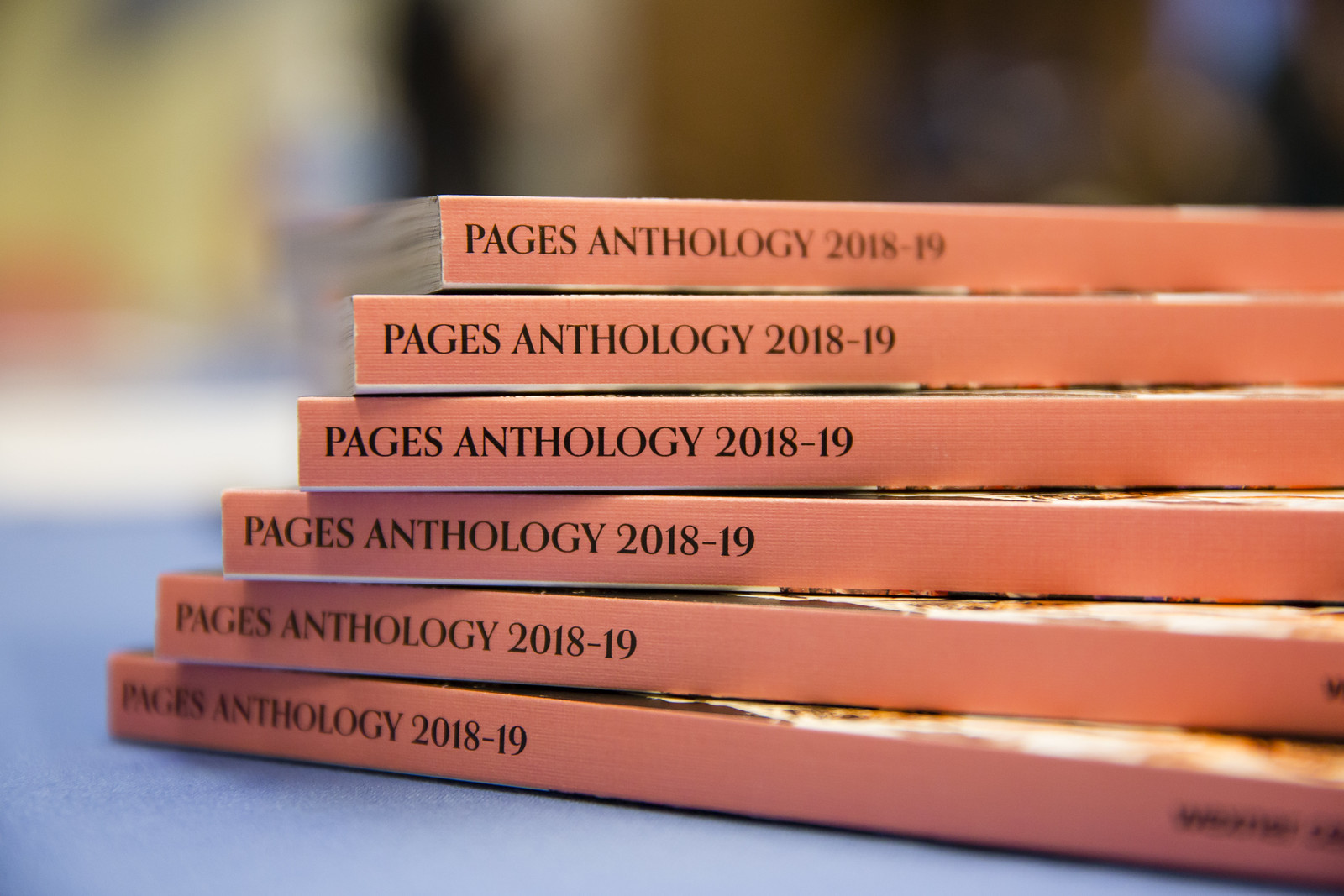A stack of six books, each titled "Pages Anthology 2018-19," is arranged in a slightly uneven, stair-like formation on a bluish tabletop. The books, which bear a pinkish, light reddish hue with black font on their spines, resemble thick magazines from past decades. Although the text "Pages Anthology 2018-19" is clearly visible at the top part of the spine, additional words near the bottom are blurred and unreadable. The background, which is also blurred, hints at a darkish classroom setting with splashes of yellow and orange colors, and possibly some brownish wooden elements.